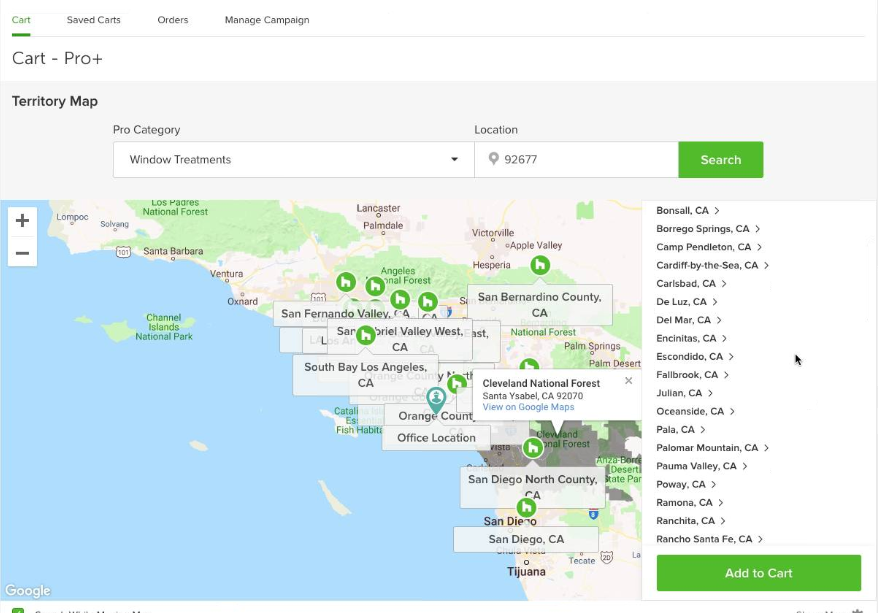**Detailed Caption:**

This is a square image. In the top left corner, bold green letters read "Cart," with adjacent text including "Saved Cart," "Orders," and "Managed Campaigns," all aligned from left to right.

Below the "Cart" section, on a white background, the text "Cart-Pro Plus" is displayed prominently. Further down, a gray banner stretches across, featuring the words "Territorium Territory Map" along with "Pro Category."

Situated beneath the banner is a search bar with placeholders for "Window Treatments" and "Location." The location field contains the value "92677" next to a pin icon. To the right of the search bar is a green button labeled "Search" in white letters.

At the center of the image, a map is visible. The ocean is on the left side, while the right side showcases several parks and multiple locations marked with green circles, each containing a white chair icon as a pin mark. Additionally, there is a prominent blue pin featuring a person icon.

To the right of the map and spanning from the top to bottom is a list within a box. The list includes place names such as:
- Bonzo, California
- Baringo Springs, California
- Camp Pendleton, California
- Cardiff by the Sea, California
- Carlsbad, California
- Del Mar, California
- Encinitas, California
- Escondido, California
- Fallbrook, California
- Julian, California
- Oceanside, California
- Pala, California
- Palomar Mountain, California
- Pauma Valley, California
- Poway, California
- Ramona, California
- Ranchita, California
- Rancho Santa Fe, California

Beneath this list, there is another green button marked "Add to Cart" in white letters.